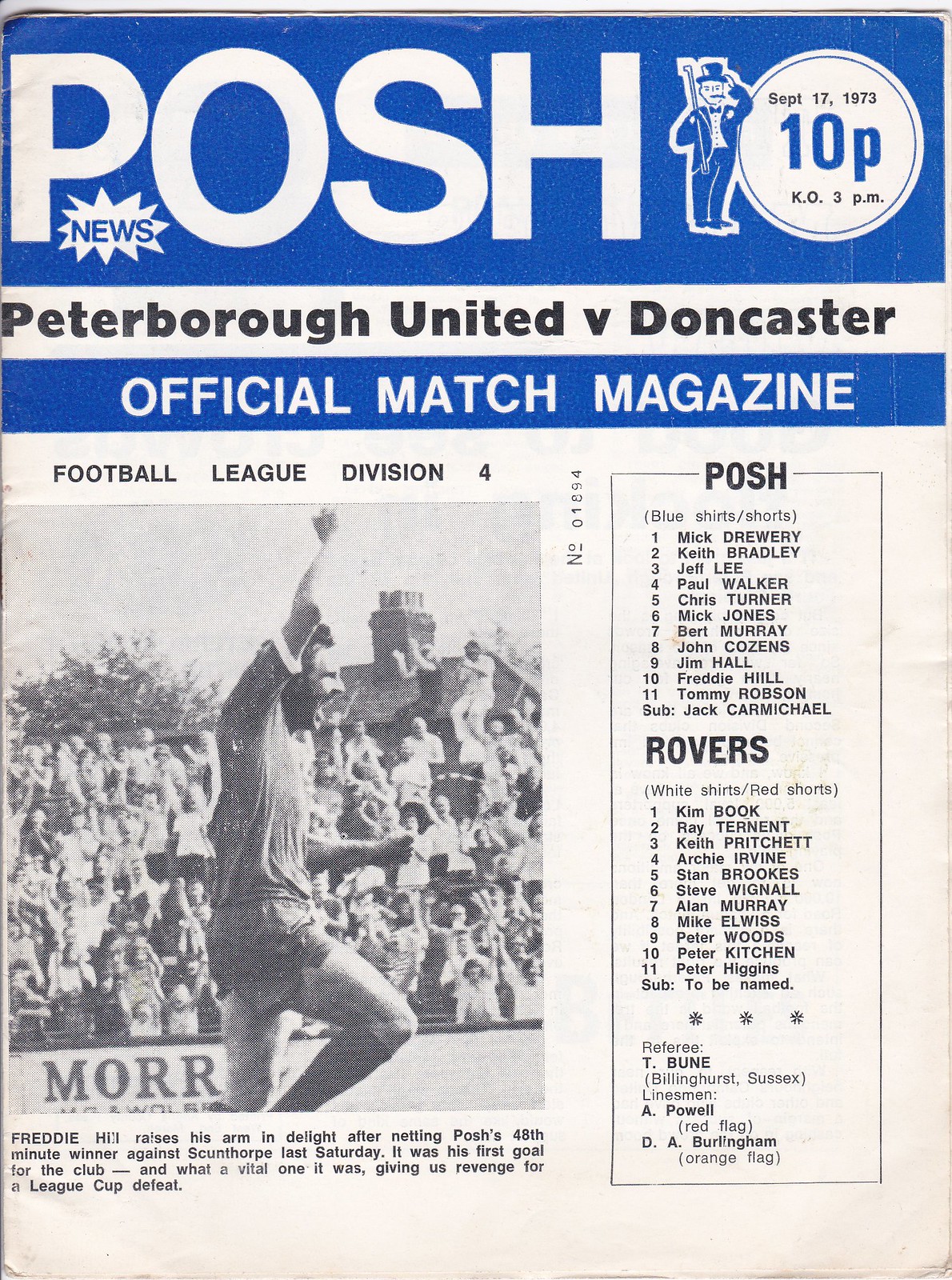The front cover of the vintage Posh catalog, dated September 17th, 1973, features an official match magazine highlighting the Peterborough United versus Doncaster game. Dominating the center is a black and white photograph of player Freddy Hill, capturing the moment he joyfully raises his arm after scoring a crucial 48th-minute winner against Scunthorpe, securing revenge for a League Cup defeat. The cover showcases large white type on a blue background with the title "POSH NEWS" beside a cartoon figure in a top hat. Below, it reads "Official Match Magazine" and details of the event timing. The left side mentions "Football League Division Four," while the right-hand side lists the team lineups, including Posh in blue shirts and shorts, and Rovers in white shirts with red shorts. The officiating referee was T. Boone Billing from Sussex, with linesmen A. Powell (red flag) and D.A. Burlingham (orange flag).